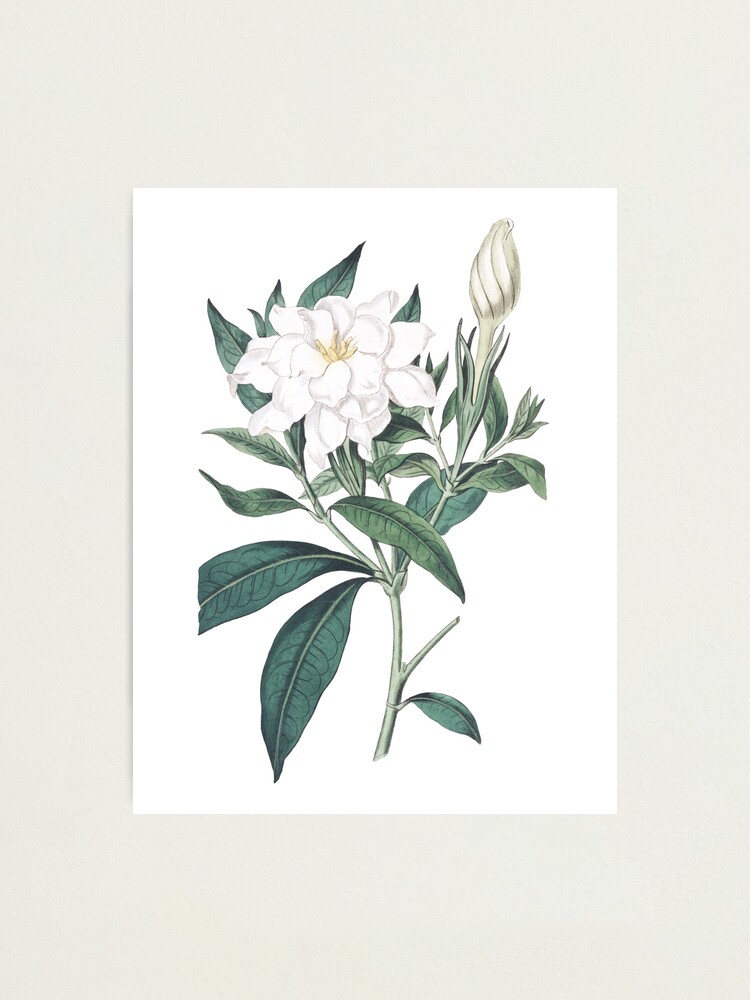This image showcases a detailed painting of a white, multi-petaled flower with yellow center stamens, which appear to be the stamen and pistils, on a branch. The painting itself has a white background and sits on a cream-colored backdrop. The flower is accompanied by long, spear-shaped, dark green leaves. To the left of the central flower, there is another bud, not yet opened, with intricate black swirly lines indicating its various layers. This unopened bud branches off towards the upper right, adding to the composition that predominantly stems upward from the bottom center and slightly branches out to the sides, creating a balanced and aesthetically pleasing visual. The overall scene resembles a white jasmine flower in its natural form.